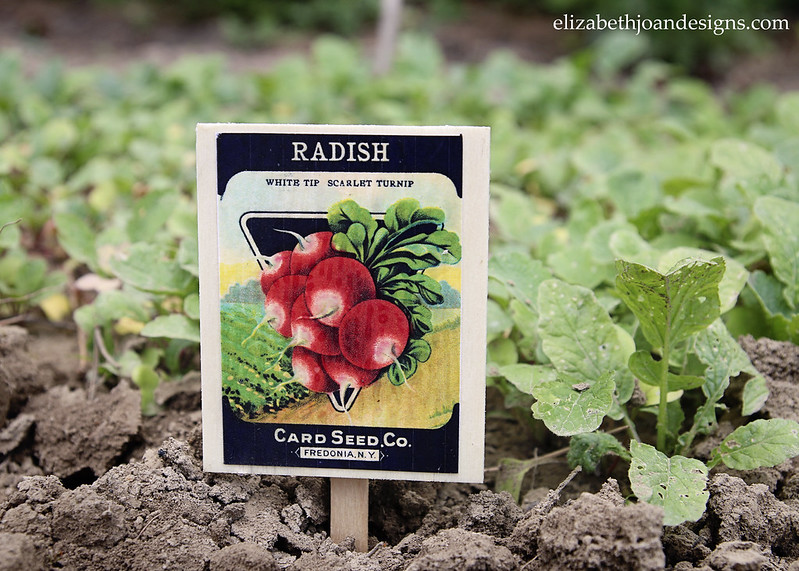The image is a close-up, horizontal photograph depicting a small section of a garden focused on a planted row of radishes. The foreground shows crumbling, light brown dirt that has been disturbed. Prominently featured is a wooden stick inserted into the ground, from which hangs a paper seed package used as a row identifier. This seed package, mounted on the stick, has a white background with a black border and contains black and white text. At the top, it reads "Radish," followed by "White Tip Scarlet Turnip" underneath. The bottom of the package specifies that it is from the "Card Seed Company" in "Fredonia, New York," with white text on a black background stating these details. Additionally, there is a painted illustration of a cluster of red and white-tipped radishes with green leafy tops on the packet.

In the garden patch, short, leafy green radish plants can be seen growing, none of which are flowering. A particularly focused radish plant to the right of the seed label exhibits some insect damage with holes in its leaves. More radish seedlings are visible in the background, albeit out of focus. The image also contains white text in the upper right corner, reading "ElizabethJoanDesigns.com," identifying the source of the photograph.